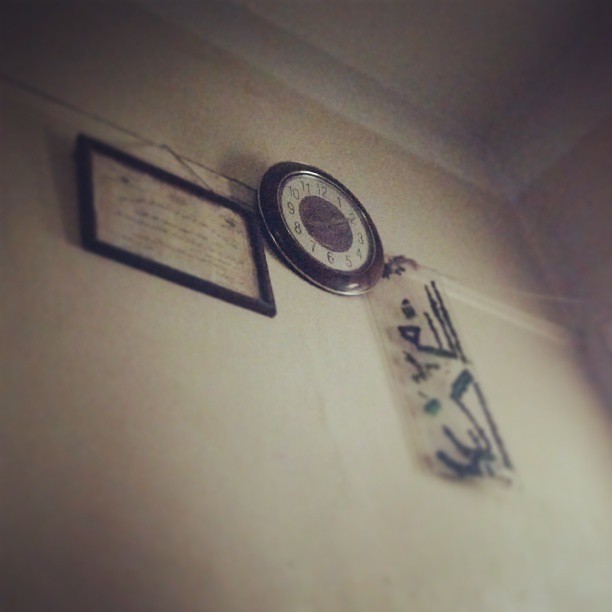This photograph captures an interior space within a building, where the perspective is angled slightly upward towards a wall. Central to the view is a round clock, encased in a decorative black frame with standard numerical indicators. Due to the blurriness of the photo, the exact time displayed on the clock is indiscernible. To the left of the clock, there is a picture frame, which appears to contain a certificate or possibly another type of formal document. The contents of the frame are not readable. On the right side of the clock, a transparent plastic item is suspended, adorned with some black markings, though their nature is unclear. The scene provides a glimpse into the wall decor and the subtle details of the surrounding environment.